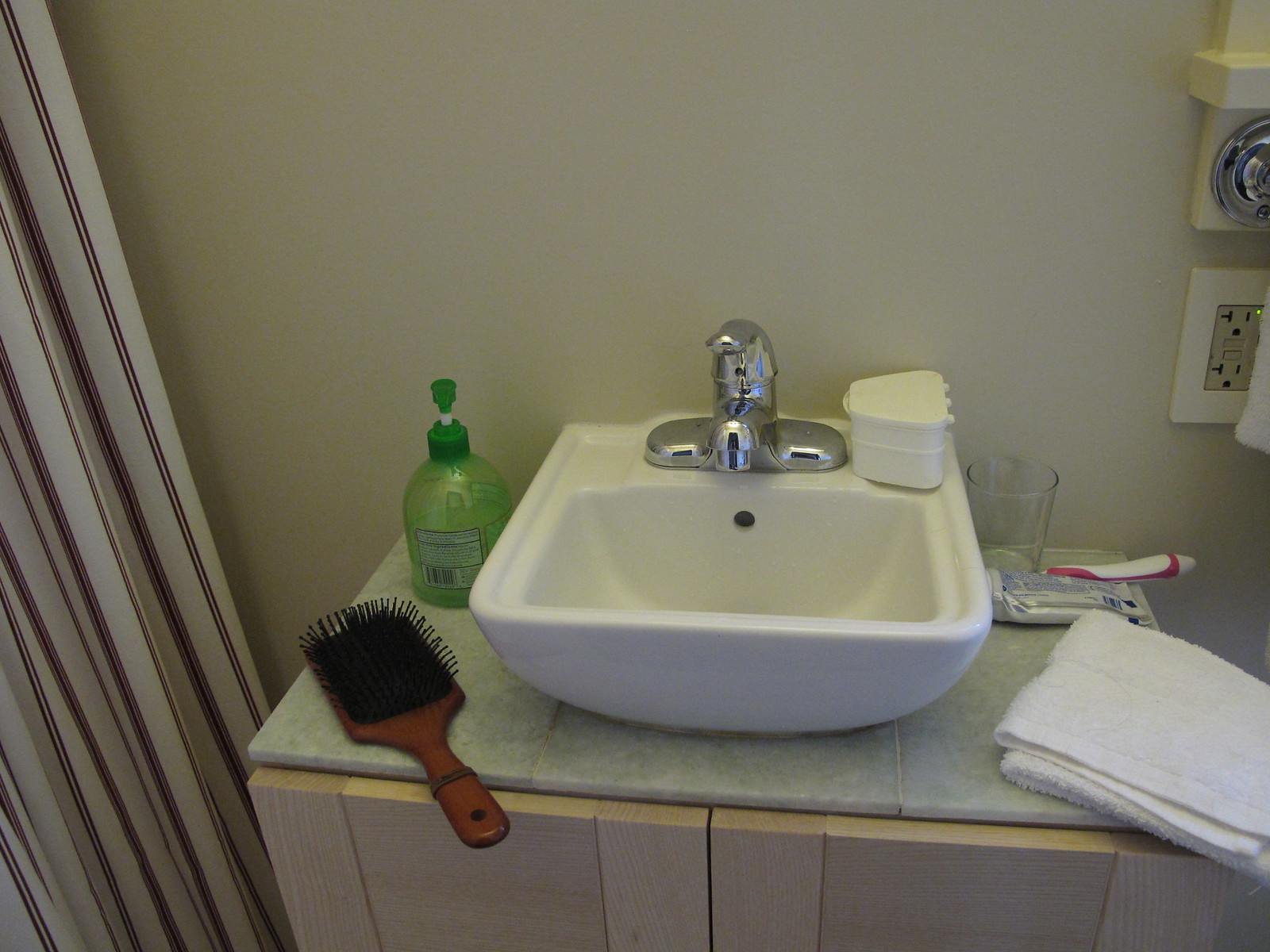The photograph captures a well-lit bathroom centered on the sink area. The sink basin is made of pristine white porcelain, complemented by a high-polished chrome faucet that gleams under the light. The sink is set into a wooden lower cabinet, crafted from light, natural-looking wood that adds a touch of warmth to the space. 

To the left side of the sink, there is a green plastic pump bottle, presumably filled with soap. Next to it, a wooden-handled hairbrush with sturdy black bristles lies on the counter, its handle wrapped with an elastic band. Perched on the sink basin is a small white container, likely used to store a retainer, mouthpiece, or tooth whitening kit.

On the right side of the sink, a clear glass stands, holding a white toothbrush and a silver tube of toothpaste beside it. A neatly folded white hand towel is also placed within easy reach, emphasizing the clean and organized nature of the space.

In the background, a cream and red striped shower curtain partially intrudes into the frame from the left, contrasting subtly against the light-colored walls. The overall atmosphere of the bathroom is one of cleanliness and order, with thoughtful placement of everyday essentials.